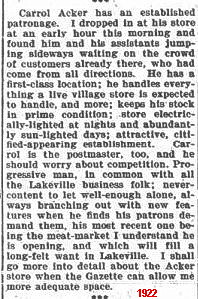The image depicts an old newspaper clipping, likely from the Gazette, characterized by black text on white paper with a small font. The article, which features at the bottom the date "1922" and a few additional marks, praises Carol Acker, a prominent business owner and the postmaster of Lakeville. The column details a visit to Acker's store early in the morning, where the author found Acker and his assistants busily attending to a large crowd of customers who had arrived from various directions. The piece highlights Acker's prime location, well-stocked inventory, and the store's attractive, modern appearance, noting it is electrically lit at night and bathed in sunlight during the day. The article describes the store as handling a wide variety of goods expected in a lively village store, and more. It also commends Acker's progressive approach to business, his readiness to innovate based on customer needs, and specifically mentions his new meat market. The writer expresses a desire to elaborate further on Acker's enterprise when more space is available.